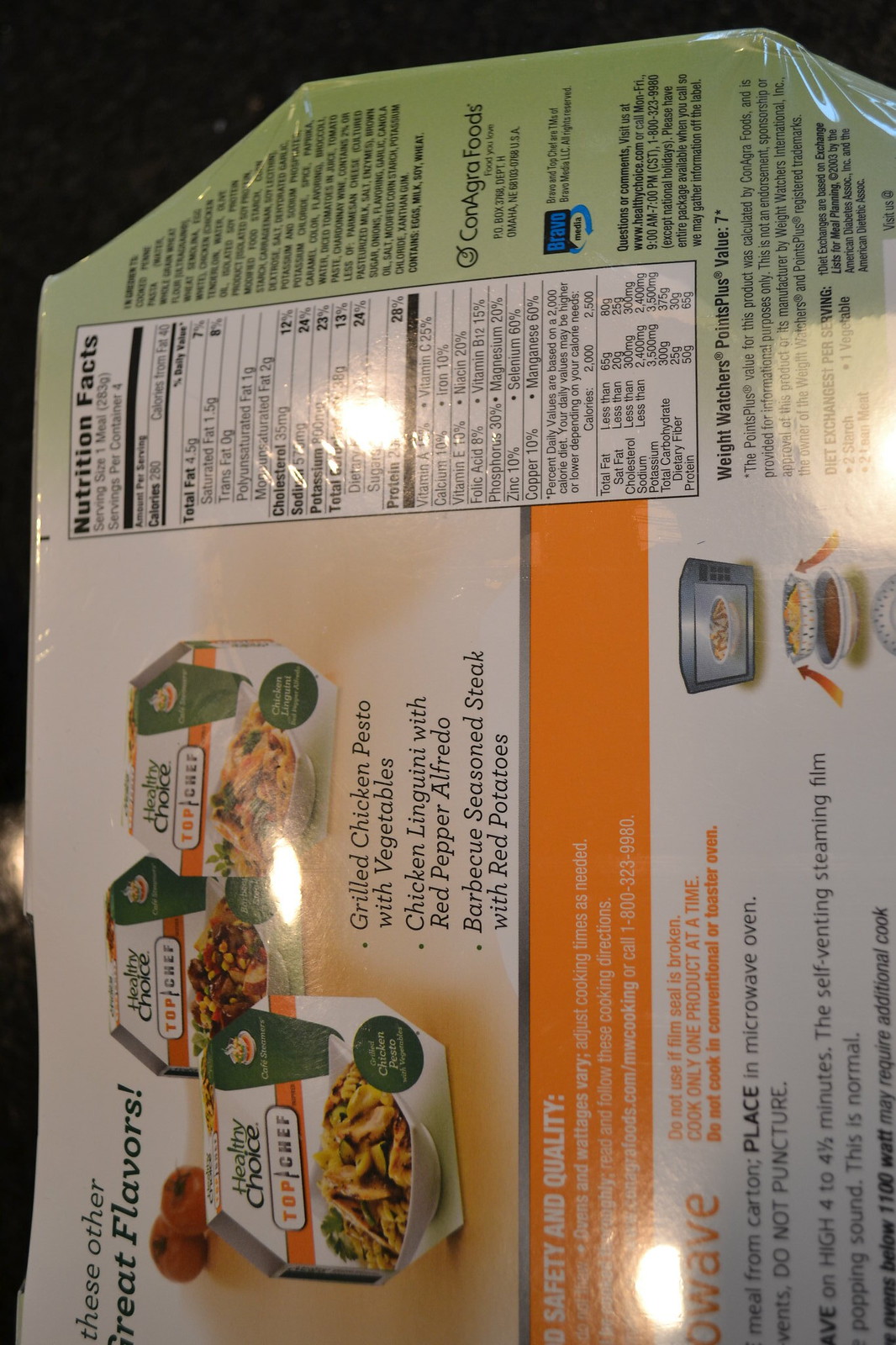This image showcases the back of a "Healthy Choice" Top Chef meal box. The box is positioned with its left side tilted towards the bottom of the screen, making the right side face the top and the top side face the left. Prominently displayed on the back are the nutrition facts, enclosed in a standard square format common to food items. Above the microwave directions, you can see three smaller images of similar meal boxes, providing a glimpse of other offerings from the same product line.